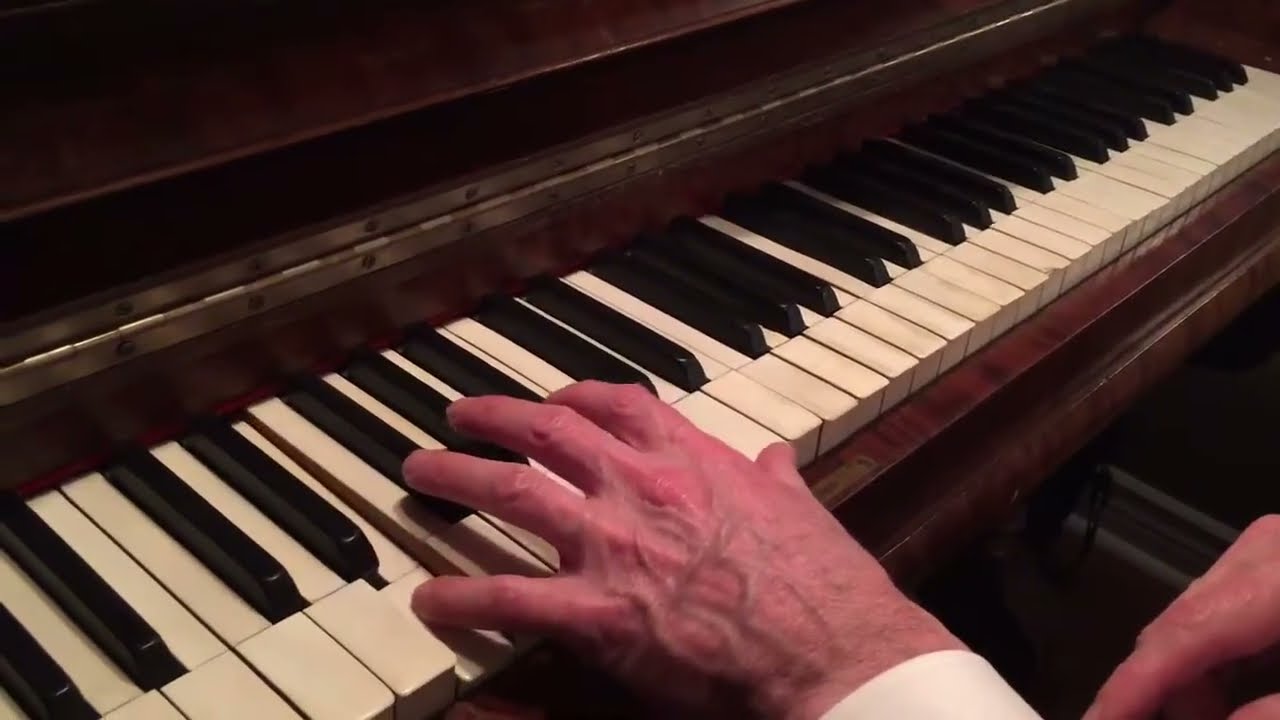The image captures a close-up of an older man’s hands poised over an aged mahogany piano. One hand, visibly veiny and slightly red, is pressing down a key with his pinky, while the other hand hovers ready to play. The piano's wooden frame, stretching from the bottom left to the upper right of the rectangular image, reveals distinct white and black keys. The man wears a white shirt, with its cuff visible on his left wrist. The scene is set indoors, focusing on the moment right before he begins to play a melody.